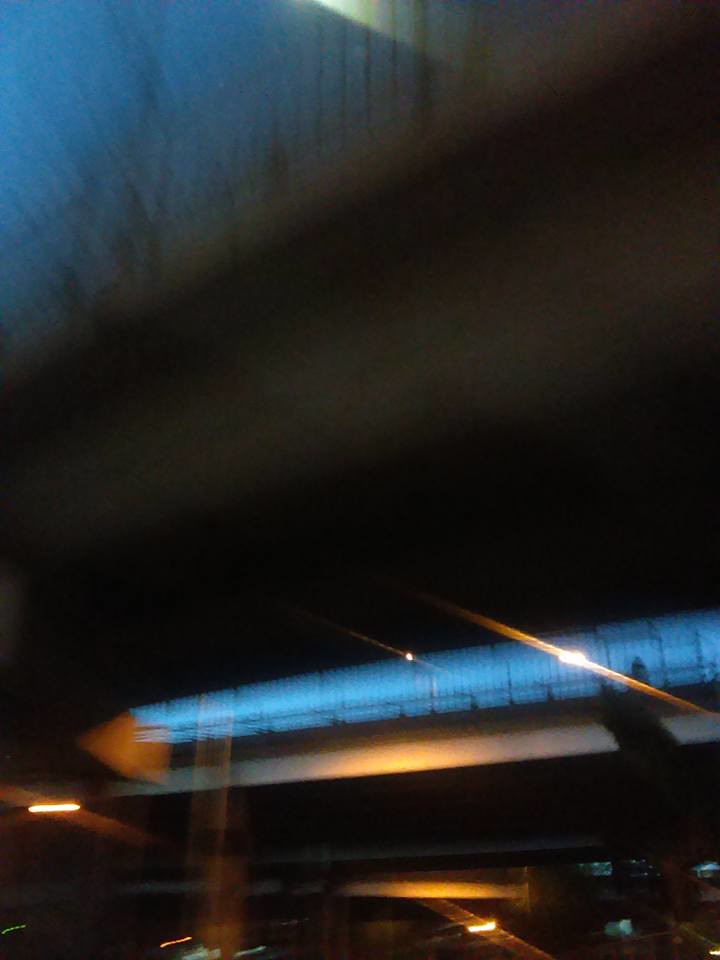The photograph is a blurry, nighttime shot taken underneath an overpass or bridge, capturing a somewhat abstract scene. The image features a central hole with a gate surrounding it, possibly for protection, hinting at an underground or parking garage location. The top of the photo displays a palette of light blue and bright blue colors, interspersed with orange and white streaks likely from streetlights, creating an overexposed effect that adds an abstract quality to the image. Diagonal lines of varying shades, from brown and tan to black, run across the photo. Additionally, there are parallel horizontal structures, resembling bridges, with noticeable bars along their sides, suggesting an intricate overhead framework. Despite the photograph's blurriness and lack of clear objects, the play of lights and lines crafts an oddly captivating scene.